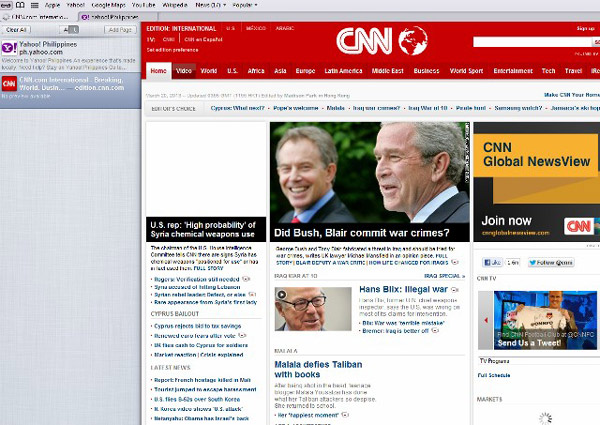This is a detailed screenshot from the CNN website viewed within an app, presenting a rather unconventional and somewhat old-school browser interface. The background features a traditional browser window, while a CNN panel appears to be floating and overlaying it. At the top, there is a bookmark bar displaying icons and options like Apple, Yahoo, Google Maps, and YouTube. The logo for Yahoo is situated on the left, followed by the CNN logo, indicating that CNN has been selected, causing its panel to pop up.

The browser itself has a retro aesthetic, unfamiliar to modern users. The CNN header is prominently displayed along with its comprehensive menu options: Home, Video, World, US, Africa, Asia, Europe, Latin America, Middle East, Business, World Sport, Entertainment, Tech, and Travel, among others.

Central to the layout is a photo of Tony Blair and George W. Bush smiling, accompanied by the provocative headline, "Did Bush and Blair commit war crimes?" Adjacent to this, on the left, a white placeholder where an image is missing contains the text, "US rep: High probability of Syria chemical weapons use," followed by various text links.

The page employs a typical three-column layout, with the central column being the widest. Here, there's mention of figures such as Hans Blix and Malala Yousafzai, with topics like "illegal war" and "Malala defies Taliban with books." To the right, a somewhat indiscernible video link or multimedia content is suggested, featuring a man holding up a shirt.